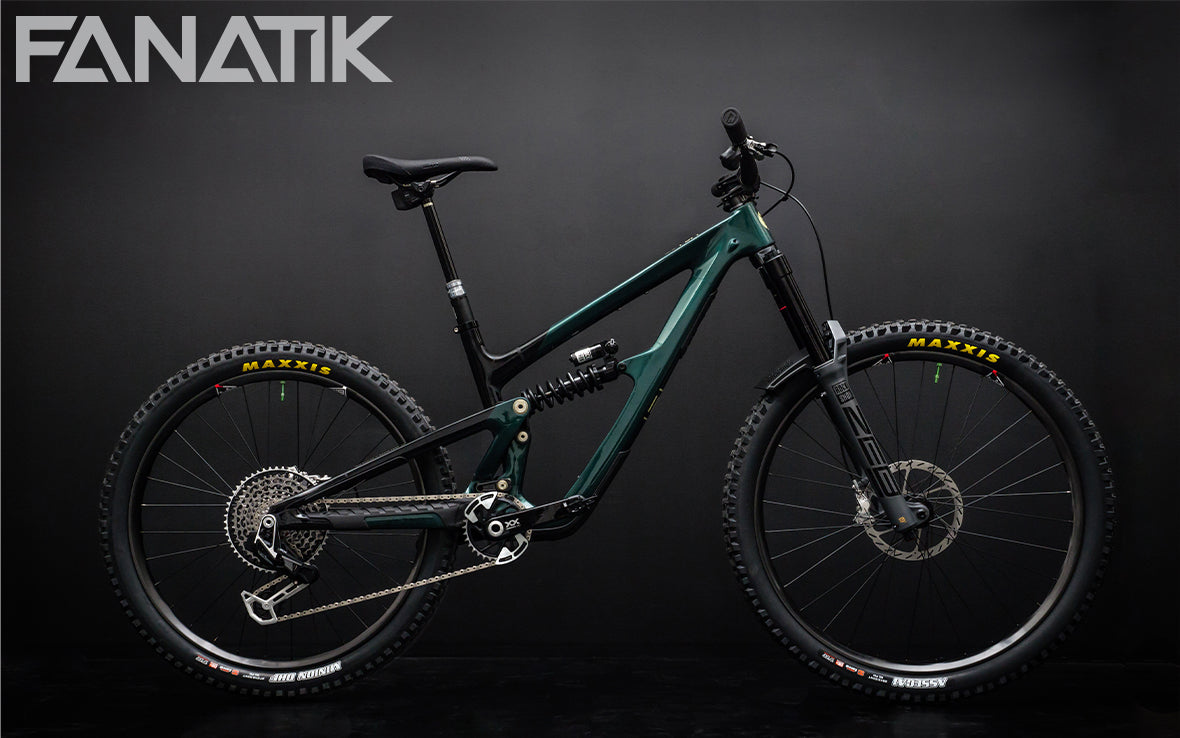This photograph showcases a sleek, futuristic bicycle set against a black and gray background, giving it a modern, almost advertisement-like appeal. Dominating the upper left corner, bold, stylized text spells out "FANATIK." The bike itself, likely a high-performance mountain bike used by serious cyclists or racers, features a dark green and black frame with a sparse design. Enhancing its aggressive look are the black tires, emblazoned with the name "MAXXIS" in striking gold letters. The tires also display various state or country flags along the bottom rim, hinting at international usage or competition. Key features include flat, straight handlebars, a high black seat, and disc brakes on the front wheel, which also appears to incorporate shock absorbers and tension springs for better shock absorption. The wheels are equipped with multiple gears, adding to the bike's intricate, advanced design. The image is framed by pitch-black borders, highlighting the bicycle's elegant, high-tech appearance.